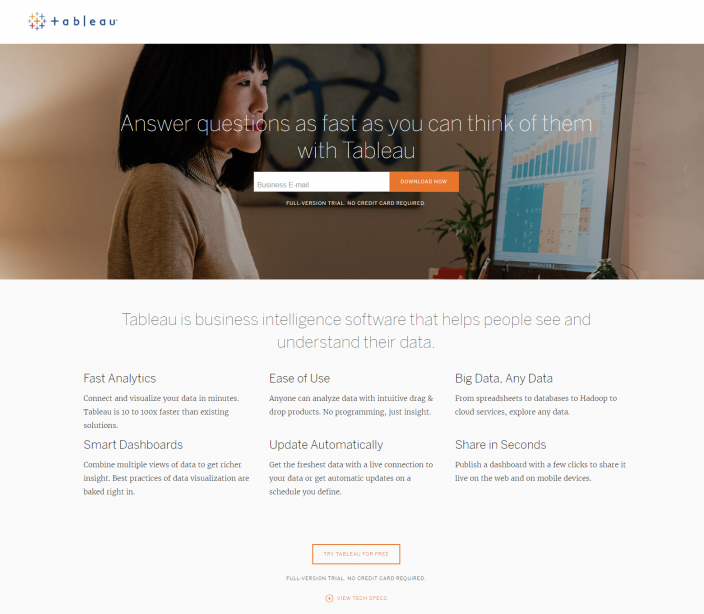The image captures a scene titled "Tableau." In the setting, a woman of Asian descent with medium-length hair and straight-across bangs is intently looking at a flat computer screen mounted against a wall. The surroundings suggest she is in her home, as indicated by a decorative photo or canvas binder on the wall. The primary focus on the screen is an interface showcasing a message in bold, white text: "Answer questions as fast as you can, think of them with Tableau." Below this, there is a prompt for entering a business email, accompanied by a prominent orange button labeled "Download it." This button offers access to a full trial version of Tableau, notably without requiring a credit card, emphasizing the convenience of exploring the full capabilities of the software without an upfront payment—unlike many trial versions which are limited.

Additionally, the screen displays an introduction to Tableau, describing it as a business intelligence software designed to help users visualize and understand their data. The description is reinforced by three informative columns:

1. **Fast Analytics**: Highlights the ability to connect and visualize data swiftly, claiming that Tableau operates ten to a thousand times faster than existing solutions.
2. **Smart Dashboards**: Stresses the capability to combine multiple data views for deeper insights, allowing for a variety of insightful analyses that update automatically.
3. **Big Data, Any Data**: Focuses on the versatility and speed of data processing and sharing.

At the bottom, a white button with an orange border invites users to "Try Tableau for free," reiterating that the full version can be accessed without a credit card. A note below reminds users to check the tech specs to ensure compatibility with their computer or laptop, ensuring a seamless installation and operation experience.